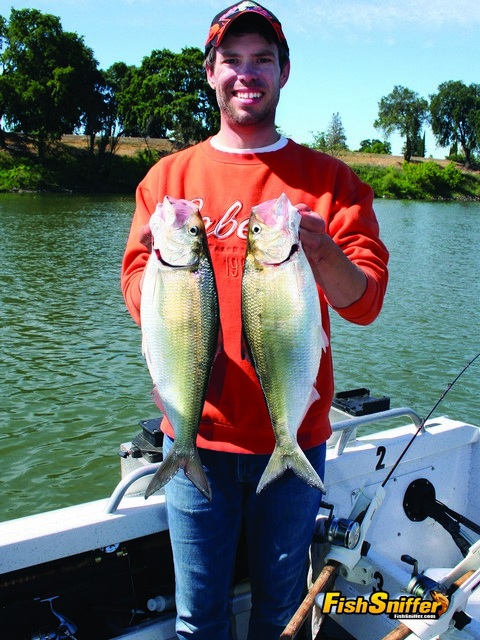A young white man in his 20s, sporting a scruffy beard, stands proudly in a boat on murky, greenish lake water, surrounded by an embankment of trees, grass, and shrubs. He’s beaming at the camera, wearing an orange shirt with partially obscured writing and an orange baseball cap. In each hand, he holds up a large fish, about three-quarters the size of his torso, gripping them by their mouths or gills. His attire, seemingly mismatched for fishing, includes blue jeans. The boat, primarily white with some black accents, has a prominent number two on it and supports a deep-sea fishing-style rigger with the fishing line still in the water. Additionally, there's writing on the bottom right corner of the image that reads "fish sniffer," potentially indicating a sponsorship or advertisement.